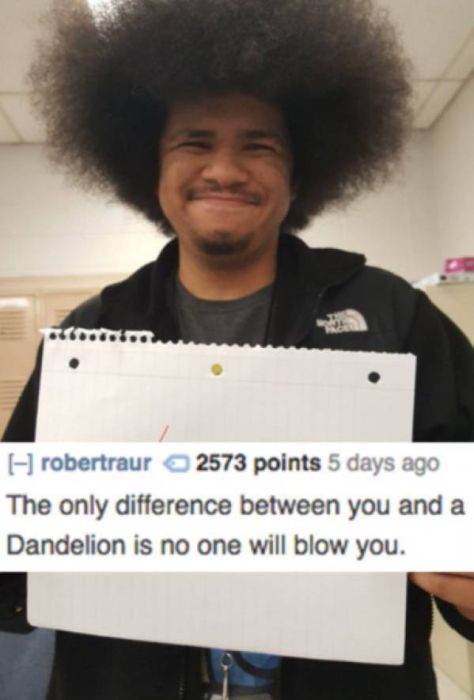The image features a young man with a large, disheveled afro, wearing a black North Face jacket over a t-shirt. He stands in what appears to be a school or locker room, characterized by a white and tan background with hints of olive, gray, and various shades of blue. The man is holding up a sheet of notebook paper, but the paper's content is obscured by a superimposed social media post. The post, which has a banner at the top, reads "2,573 points · five days ago" and continues with the text: "The only difference between you and a dandelion is no one will blow you." The young man wears a goofy smile as he poses, making the entire scene resemble a meme typically found on platforms like Reddit or Twitter. The overall composition is centered, with the focus being on the playful yet slightly mocking tone of the meme text layered over the photo.